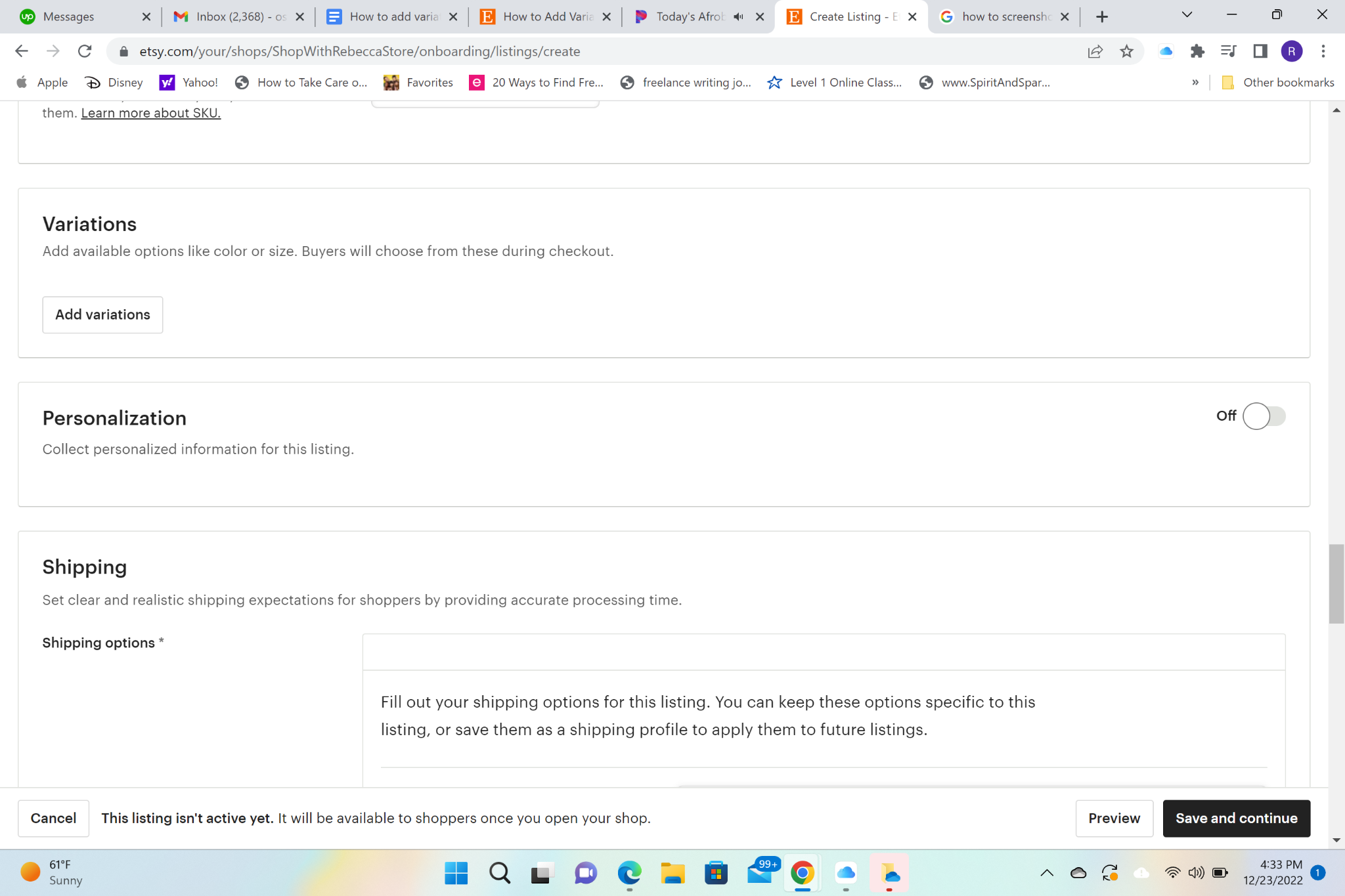Here is a detailed and descriptive caption for the provided image:

---

This screenshot captures a browser window focused on an Etsy page. At the top of the browser, seven tabs are open, with the second to last tab being the active one. The URL bar clearly displays "Etsy.com." Beneath the URL bar, there is a bookmark bar featuring nine favorited links: Apple, Disney, Yahoo, "How to Take Care," "Cutoff," "Favorites," "20 Ways to Find Something," "Freelance Writing," "Level One Online Class," and "Spirit and Spar..." Below the bookmark bar, the Etsy page itself is divided into three main sections: Variations, Personalization, and Shipping. The Personalization section features a toggle button on its right side, while the Variations section contains a button labeled "Add Variations" underneath it. The clean, white background of the page highlights these sections clearly, displaying a structured interface for easy navigation and customization.

---